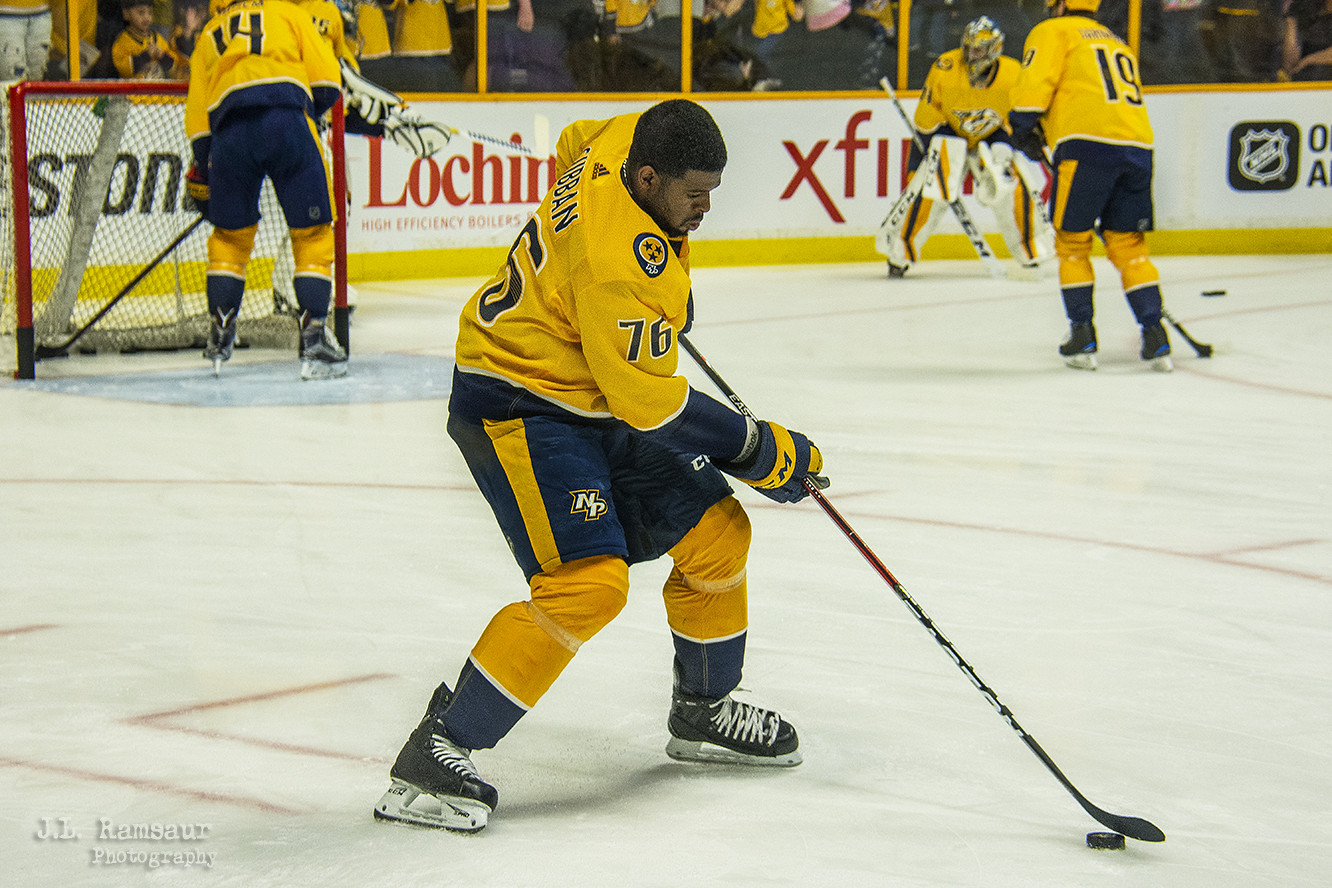This is a photo capturing what appears to be PK Subban, number 76, in the midst of a live hockey game, positioned at the center of a brightly lit rink. Subban, identifiable by his distinctive golden-yellow jersey adorned with dark blue accents and matching dark blue shorts with yellow trim, is intensely focused as he maneuvers a black hockey stick towards a puck lying on the ice near the bottom right corner of the image. Surrounding him are four other players, also clad in similar uniforms, including players numbered 14 and 19. In the upper left background, the goalie is near the red goalpost, with another player approaching. The backdrop reveals a glass wall with spectators eagerly watching the game. Further enhancing the image’s professional composition, the bottom left corner features the text "JL Ramsar Photography."